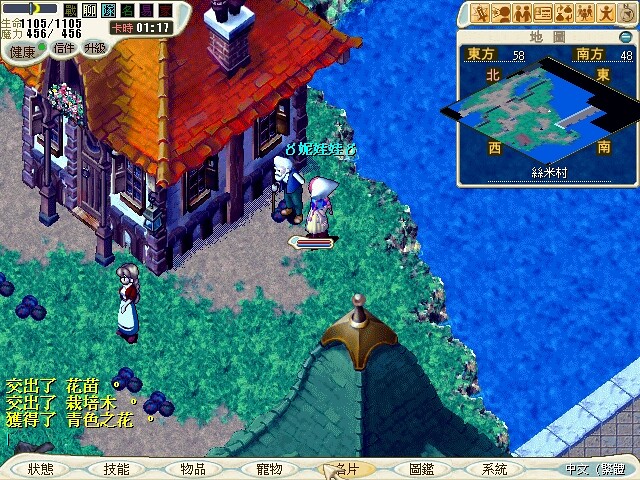This captivating screen capture from an unknown video game showcases a dazzling, animated scene rich with detail and vibrant colors. The backdrop features a picturesque village with older, charming houses adorned with chimneys and tiled roofs, complemented by sturdy brick and stone walls. Verdant grass and serene water bodies add to the tranquil setting, while all textual overlays appear in an unidentified Asian script.

In the foreground, three distinctly animated characters take center stage. On the left, an elderly man with flowing white hair and a beard stands, exuding wisdom and experience. To his right, a woman donning an elaborate, oversized bonnet conceals most of her features, adding an air of mystery. Next to her, another woman, distinguished by her long blonde braided hair and traditional skirt, brings a touch of rustic elegance to the scene. The overall image is a feast for the eyes, meticulously detailed and alive with storytelling potential.